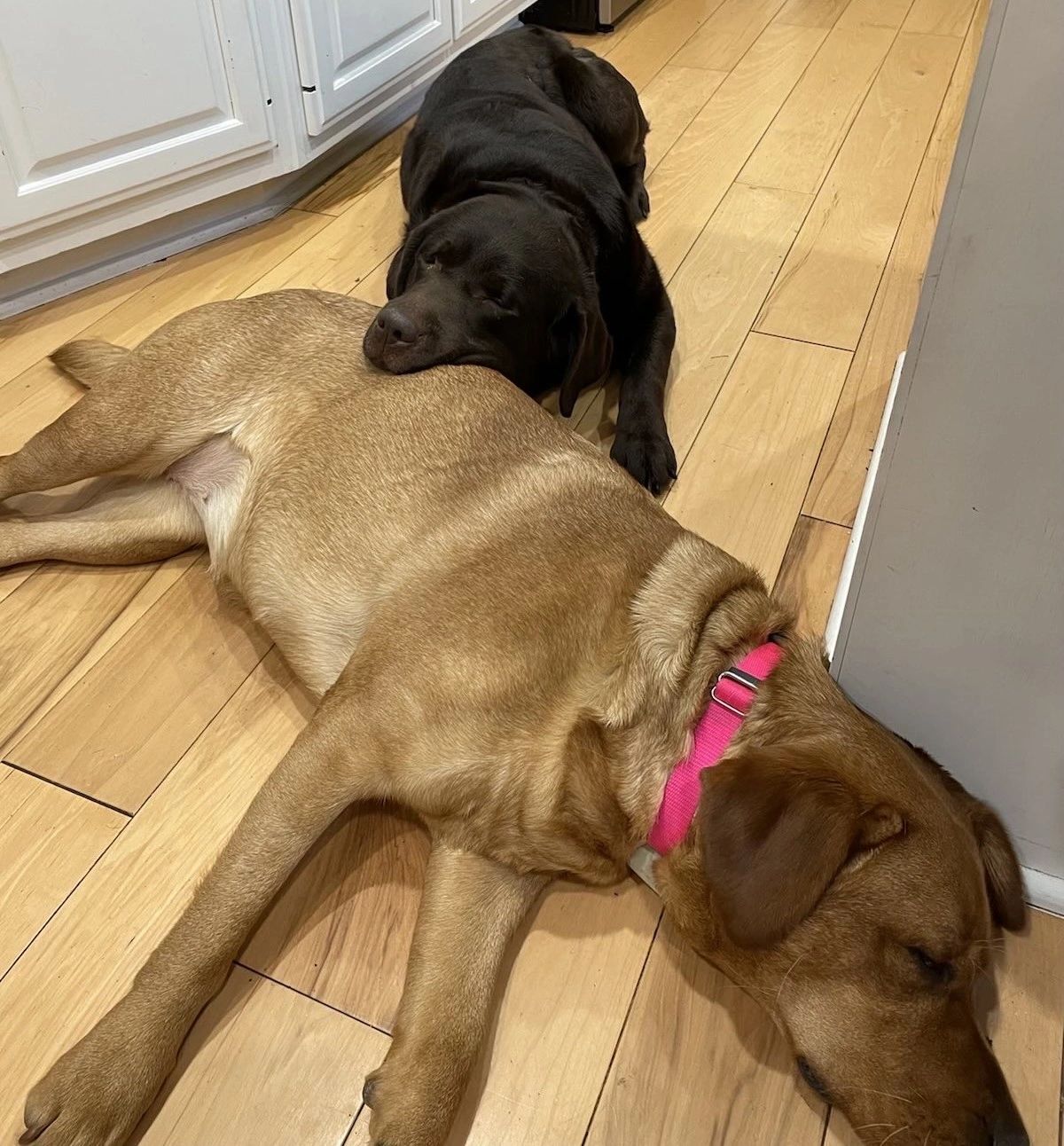The image depicts two Labrador-type dogs resting peacefully on a pale, wooden kitchen floor. The dog in the foreground is a golden brown hue with a muscular, lean physique and is adorned with a pink collar. This dog lies on its side with eyes closed, stretching across approximately 75% of the image, its head positioned toward the lower right corner. Behind it, a sleek black Labrador rests its head on the golden dog's rear, lying on its belly. The black dog blends into the background due to its dark fur but appears equally at ease, possibly asleep. The background reveals a glimpse of white cabinetry on the upper left and a taupe wall on the right side of the image, suggesting the scene is set in a kitchen or hallway. A black object, potentially a washing machine or refrigerator, extends from the cabinets. Both dogs exude an aura of tranquility as they lay sprawled out on the wood floor, their soft and short fur catching faint, natural light.